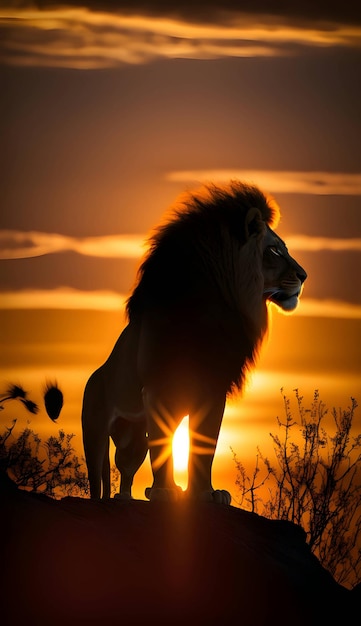Against a backdrop reminiscent of a Lion King scene, a majestic male lion stands boldly on the edge of a boulder, his silhouette sharply defined by the setting or rising sun. The sun's rays pierce through the open space between his strong front legs, casting a brilliant orange glow that envelops the scene. His flowing mane catches the light, creating a halo effect around his powerful frame. The lion faces to the right, his profile dominated by a darker face and a strikingly white chin. Thin, horizontal clouds stretch across the sky, bathed in warm, golden hues, while wispy plants frame the rocky outcrop both to the left and right. Despite the darker tones prevailing in the photograph, the sun's illumination delineates the lion's form, emphasizing his grandeur and the rugged, natural beauty of his surroundings.